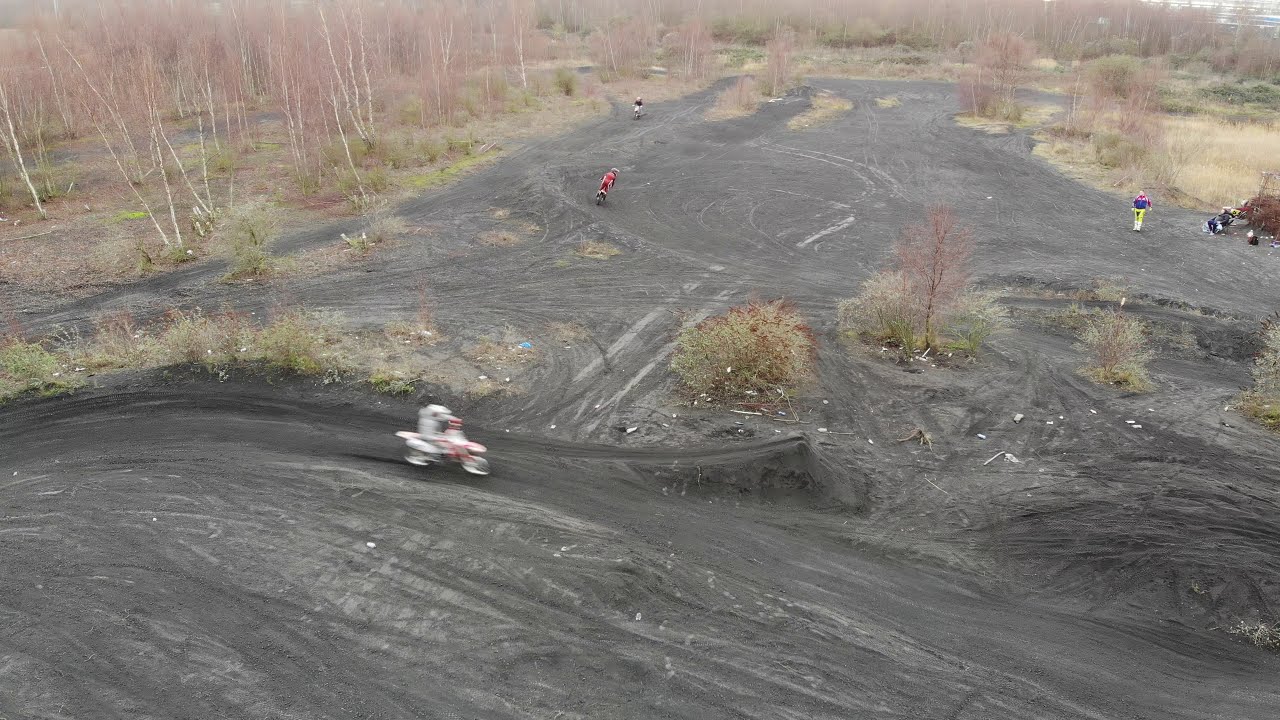In this image, we see a sprawling outdoor dirt bike track with a grayish-brown dirt terrain, crisscrossed by numerous tire tracks. Dominating the foreground is a blurred, white dirt bike mid-motion, capturing the essence of speed. Close behind, another rider in a red outfit is visible, further adding to the dynamic activity of the scene. A third dirt bike rider is faintly discernible in the distance. On the right side of the image, a man in yellow pants and a blue shirt stands as an observer. Surrounding the track, the landscape features scattered, leafless trees with white bark and patches of dry, brownish grass. The backdrop is a blend of more barren trees and hints of what might be a distant water body, adding depth to the setting. The image is purely focused on the lively dirt bike arena and the natural surroundings, devoid of any text or sky.